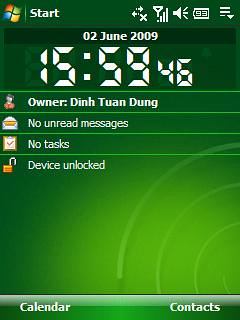This image appears to be a computer-generated screenshot of a mobile-friendly version of a Windows desktop interface. The screen has a green background with white text. At the top left corner, there's the Windows logo accompanied by the word "Start." Along the upper section, there are several icons, likely representing different applications or system functions.

The interface also displays a time and date stamp prominently, suggesting this image captures a specific moment in time. Below the time and date, a list of application icons is organized vertically. These include icons related to emails, tasks, and a key-like icon labeled "Device Unlocked," indicating the device's current status.

Towards the bottom of the screen, two distinct icons labeled "Calendar" and "Contacts" are visible, likely providing quick access to these essential applications. The overall layout is reminiscent of a simplified, touch-friendly version of a traditional Windows desktop, tailored for mobile device usage.